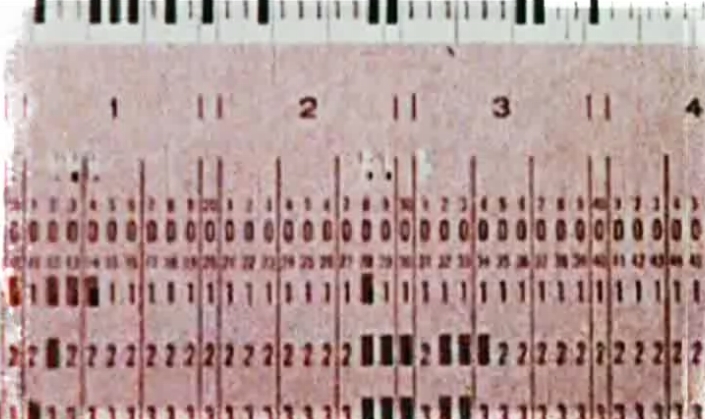This close-up photograph depicts a weathered, yellowish-pink sheet of paper that appears to be some sort of scaled measurement device reminiscent of a ruler. The paper is marked with evenly spaced numbers 1, 2, 3, and 4 from left to right, though the sequence is cut off after the number 4. Each number is framed by two vertical bars on both its left and right sides, with additional small lines and markers occupying the spaces between these bars. Below each numeric section, there are long vertical dashes and multiple rows of shorter horizontal lines, which exhibit patterns of repetition in thickness and spacing. The rows include sequences of numbers and small bars, albeit with no immediately recognizable pattern. The color scheme includes pinkish hues for the background, with text and lines primarily in black and some in dark red or purple. The paper's upper section bears resemblance to the bottom half of piano keys, adding to the intricate details of the image.